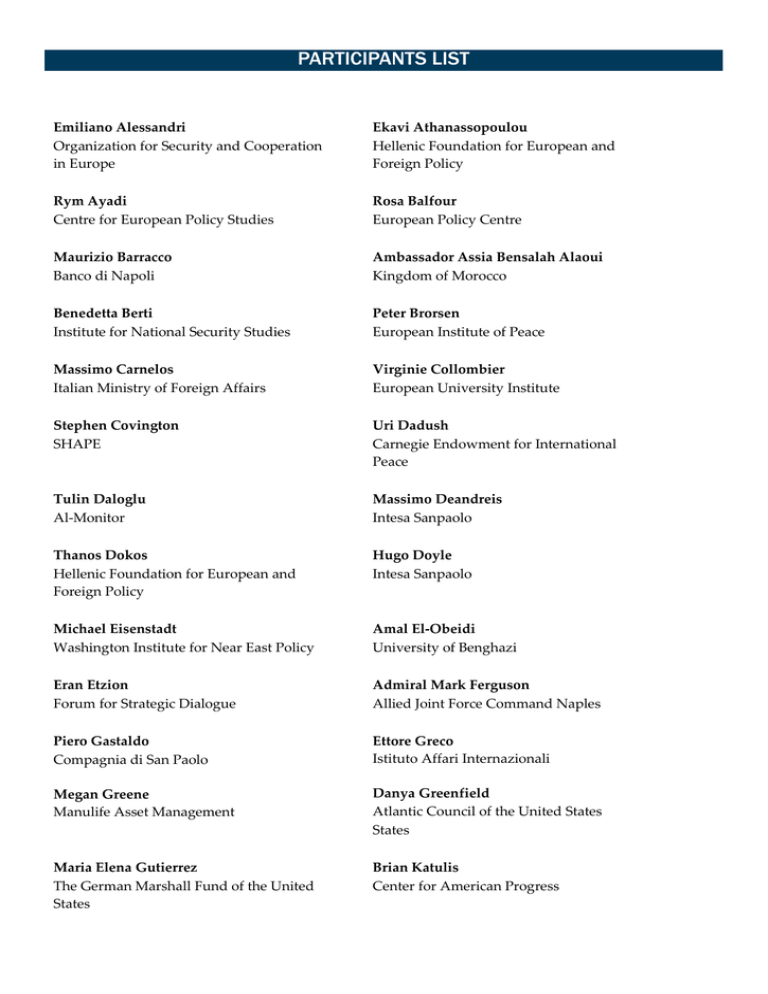The image showcases a structured participation list, prominently featuring a black rectangle at the top that bears the title "PARTICIPATION LIST" in bold white, all-caps lettering. Below this header, two columns display a meticulously organized compilation of names and their corresponding affiliations.

On the left column, names such as Emiliano, Alexandra, Rem, Aodai, and Stephen Covington are presented in bold black letters. Each name is promptly followed by a secondary line specifying their respective organizations or regions. For instance, Stephen Covington's affiliation is clearly noted beneath his name.

Similarly, the right column follows the same formatting. The bold black names include individuals like Rosa Balfour, who is identified as being from the European Policy Center. Another entry in this column lists an Ambassador—accompanied by a name that is not easily pronounceable—from the Kingdom of Morocco. This systematic, two-column format neatly categorizes participants and their affiliations, ensuring clarity and ease of reading.